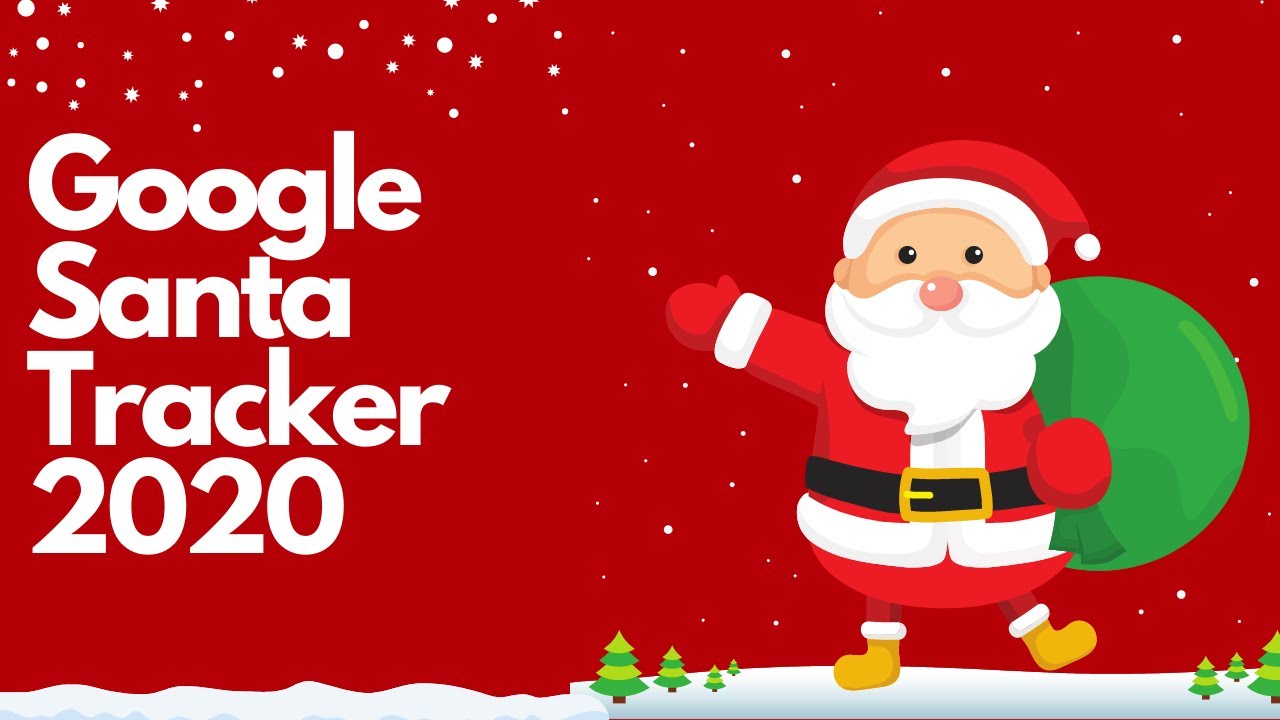A vibrant digital advertisement for the Google Santa Tracker 2020 features a festive rectangular screenshot with a bright red background and delicate white snowflakes gently falling throughout the scene. The snowflakes are dispersed except for a notable gap on the lower left-hand side, extending up to about 75% of the image. Within this area, four lines of white text prominently display "Google Santa Tracker 2020," each word occupying its own line.

At the bottom of the screenshot, a snowy landscape extends across the scene, dotted with small, festive Christmas trees concentrated towards the right side. Dominating the right side of the image is a jovial depiction of Santa Claus, taking up roughly 75% of the picture space. Santa is clad in his iconic red coat, matching red pants, tan boots, red gloves, and a red and white hat. His cheerful face is framed by a large white beard, and he exudes holiday cheer with one arm raised in a friendly wave. In his other hand, he firmly grasps a large green sack, symbolizing the bag of gifts he plans to deliver. This image encapsulates the spirit of the holiday season, combining traditional Christmas elements with the modern touch of Google's interactive Santa Tracker.